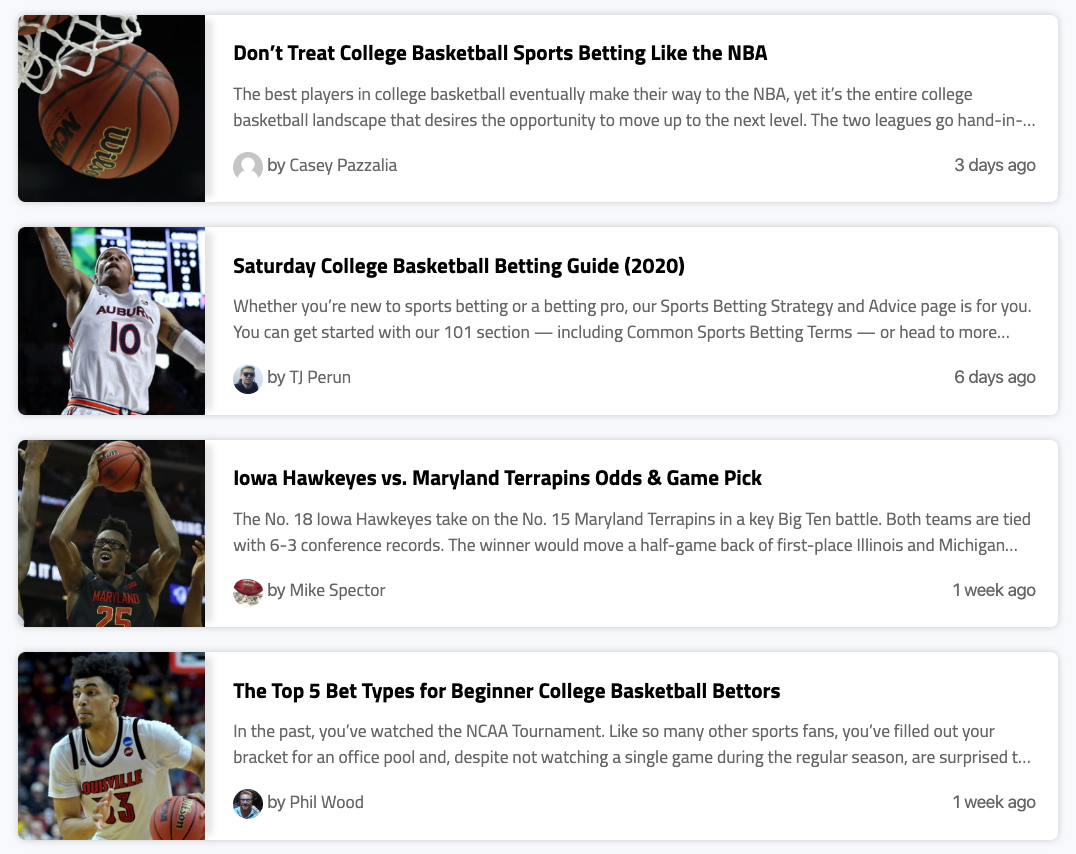This image is a screenshot depicting a collection of sports stories displayed in a vertically scrolling format. Each story is presented within a horizontal white box, arranged vertically down the gray background of the page. 

At the top left, there is a prominent thumbnail image featuring a basketball going through a hoop. Adjacent to this thumbnail, on the right, is the headline for the featured story: "Don't Treat College Basketball Sports Betting Like the NBA." Beneath this headline is a brief teaser that states, "The best players in college basketball eventually make their way to the NBA, yet it's the entire college basketball landscape that desires the opportunity to move up to the next level." The teaser ends abruptly, inviting users to click through to read the full story.

In the bottom right corner of the top story box, there is a user profile photo. Next to it, the author's name, Casey Pozzuola, is displayed, along with the posting date which indicates the article was published three days ago.

Following the same format, subsequent sports stories are listed below: each has a thumbnail image on the left, the article title at the top, the author's name in the bottom left, and the posting date in the bottom right.